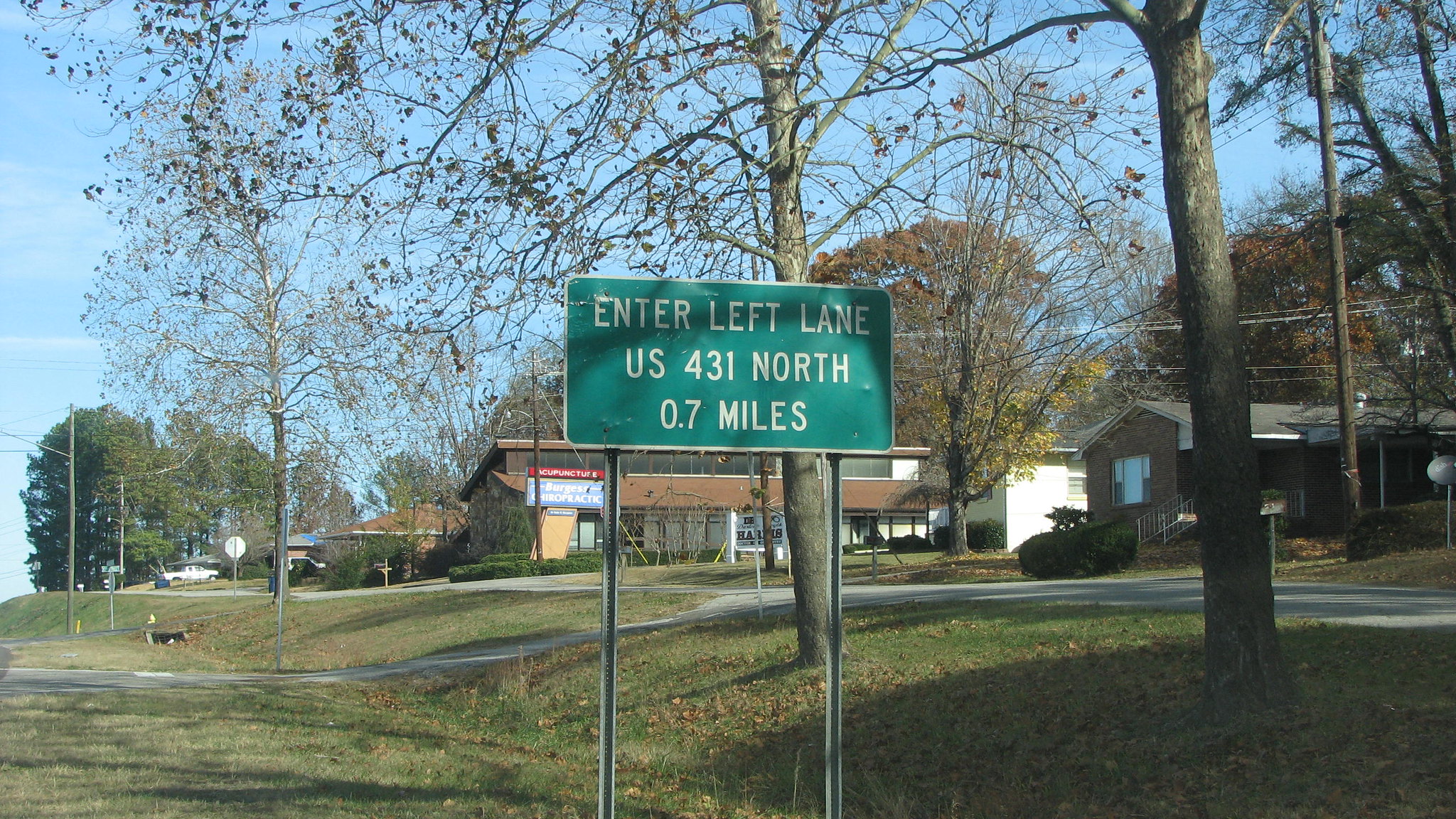The image prominently displays a green road sign with a white border and rounded corners. The sign reads, in white block letters: "Capital, Inter-Left Lane, U.S. 431 North, 0.7 miles." The sign is mounted on two gray posts, which could be made of either galvanized metal or stainless steel. 

In the background, there is a lush green lawn, a driveway possibly leading to a street, and a variety of trees. There are also street lamps and the back of a stop sign visible. Several structures line the street, including what appear to be both houses and businesses, one of which is identified by a sign close to it. The setting suggests the sign is on or near a highway, though the highway itself is not visible in the image.